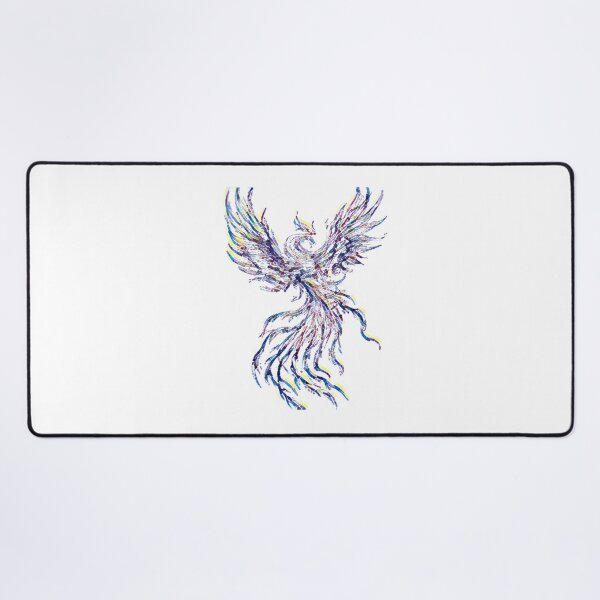The image is an intricate illustration of a phoenix, placed centrally within a rectangular frame bordered by a thin black outline. The phoenix, though relatively small, captures attention with its dynamic, feathery appearance, suggesting it was drawn with either colored pencils or fine ink-like pens. Though its face blends somewhat with the background due to the style and size, the bird itself displays a stunning array of colors, creating a rainbow-like effect with shades of blue, purple, pink, yellow, green, and orange. The background is a light grey, further highlighting the vibrant hues of the phoenix. Its wings are spread wide in mid-flight, with long, colorful feathers extending to a similarly multi-hued tail. Despite its detailed plumage, the phoenix also features dragon-like characteristics, such as horns, legs, and hooves, inviting a fascinating blend of mythological elements into the artwork.